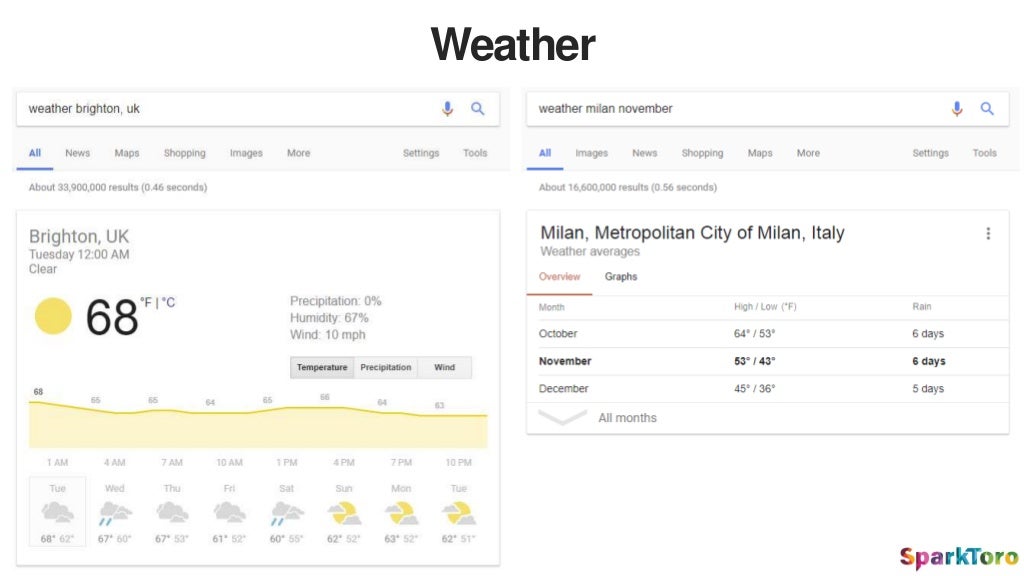The image is a screenshot set against a plain white background, showcasing a weather update interface. Dominating the center, in large, bold black text, is the word "Weather." Positioned in the upper left corner within a white search bar are the words "Weather Brighton UK," accompanied by the Google microphone icon and a magnifying glass icon, indicative of search functionality. 

Below the search bar, spanning from left to right in a gray box, are navigational options: "All," "News," "Maps," "Shopping," "Images," "More," "Settings," and "Tools." 

In a separate section outlined in gray, located in the upper left corner, is a detailed weather report for Brighton, UK. It specifies that the update is for Tuesday at 12 a.m., describing the weather as clear. A bright yellow sun icon symbolizes the clear conditions. The temperature is displayed prominently as 68 degrees Fahrenheit. Additional weather details include 0% precipitation, 67% humidity, and 10 miles per hour wind speed.